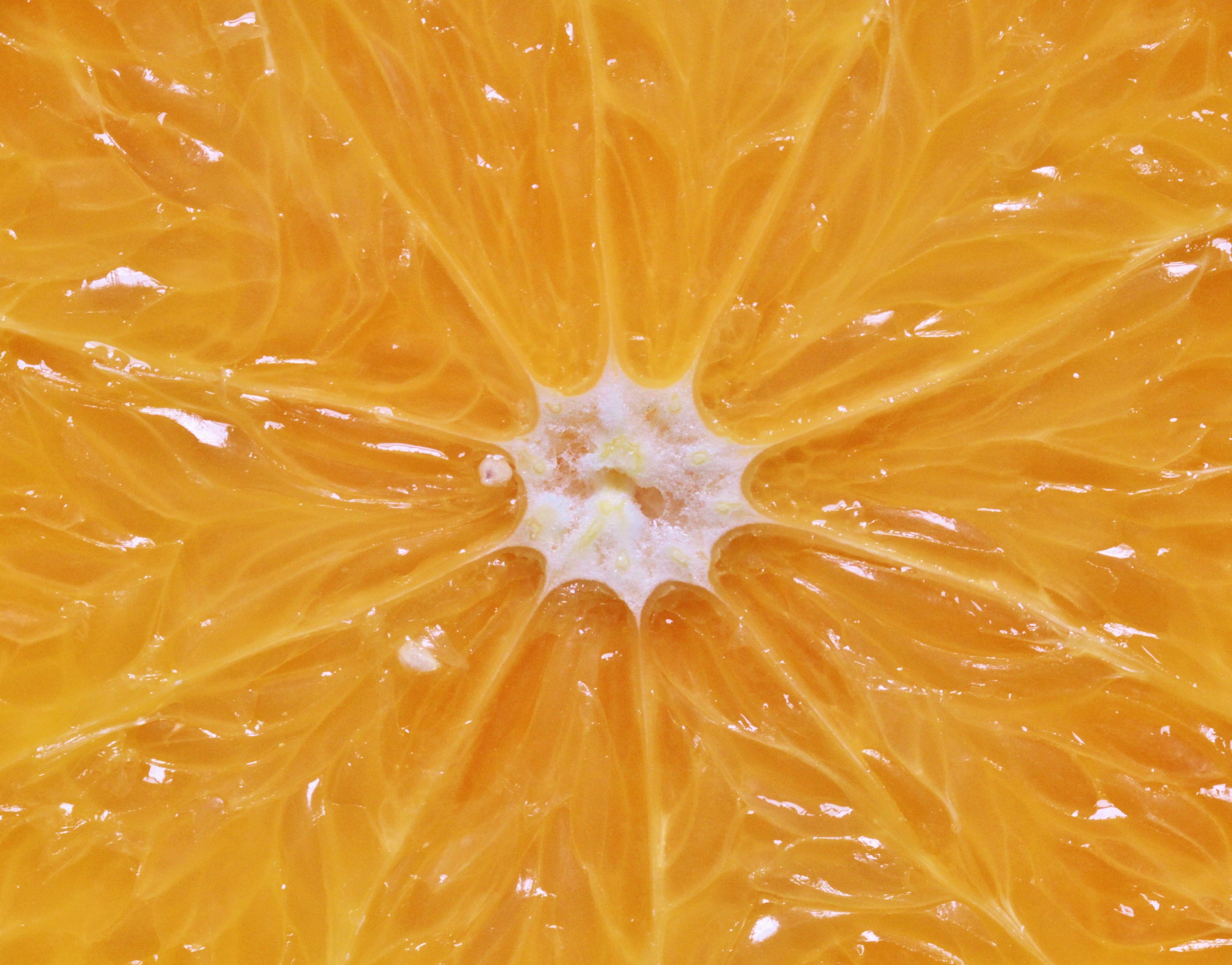This image presents a highly detailed, close-up view of the interior of an orange, focusing on the intricate structure at its center. The composition features a starburst pattern emerging from a distinct central white area, reminiscent of a ten-sided star or a volcano's sharp, radiant points. Extending from this white center are orange segments, arranged like soft, pulpy tentacles that radiate outward, highlighting the juicy, bright orange flesh. The segments are depicted in a triangular form, sliced midsection to reveal the rich, textured pulp without showing the outer peel. Light reflections on the surface add a sense of freshness and depth to the vibrant scene, enhancing the juicy appearance of this tightly framed shot, approximately two inches wide.